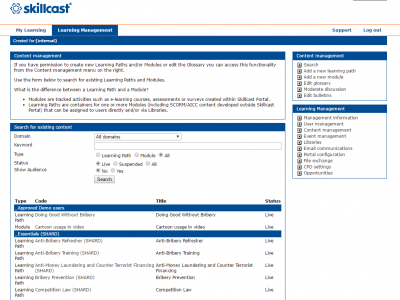This image is a screenshot of the Skillcast webpage, presented in a square format and centered on the screen. In the upper left-hand corner of the screenshot, a distinctive blue, almost floral-shaped logo is prominently displayed. Adjacent to this logo, the brand name "Skillcast" is boldly printed in a deep blue font, providing immediate brand recognition.

The webpage layout is meticulously structured, divided into several distinct sections. At the top of the page, there is a rectangular section, followed by a square section positioned at the lower left-hand corner. Additionally, there are two more square sections located in the upper right.

Each of these sections features black text, although the text is not legible in the screenshot. A consistent design element across these sections is a blue banner that spans horizontally at the top of each one, tying the design together cohesively. The overall layout is clean and organized, reflecting a professional web design.